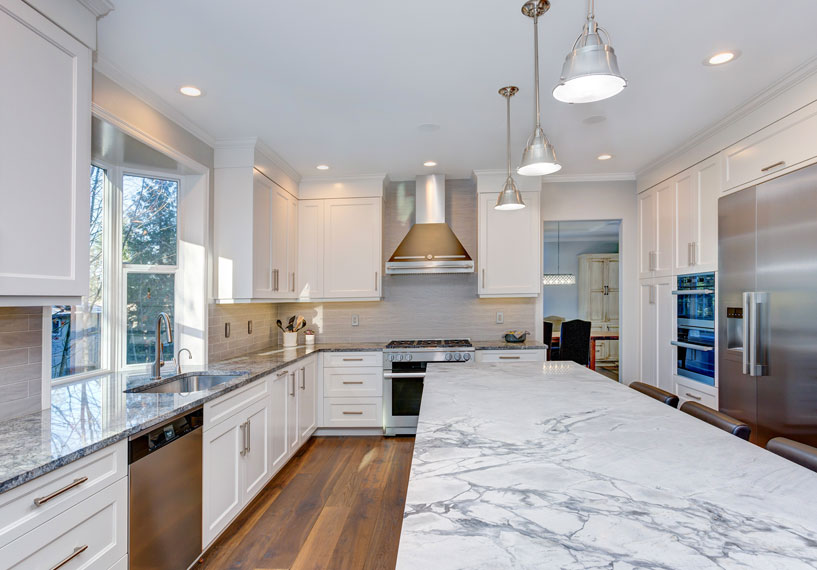This image showcases an immaculate and modern kitchen characterized by its bright, clean aesthetic. The kitchen features a striking contrast between its white ceiling, off-white cabinetry, and the cohesive gray-and-white granite countertops. The countertops extend along the left wall and form a prominent island on the right, with three brown leather bar stools neatly aligned beside it.

The island, topped with the same luxurious stone, is illuminated by three sleek, metallic silver pendant lights hanging from the ceiling. Additional recessed lighting further enhances the kitchen's brightness. The floor is a warm, polished wood, adding a touch of natural coziness to the space.

On the left side of the image, a stainless steel dishwasher is positioned below the counter near a bay window. The window allows natural light to flood in, complementing the room's recessed lights. The countertop here also includes a sink, perfectly situated beneath the window.

Towards the back of the kitchen, a stainless steel range and a shiny metal hood form a focal point in the design, surrounded by ample cabinetry. Just to the right of the island, the kitchen boasts a towering double-door stainless steel refrigerator. Adjacent to it, there's a pair of stacked convection ovens or microwaves, integrated seamlessly with the surrounding white cabinets.

Overall, this kitchen is both highly functional and visually pristine, with an elegant blend of stainless steel appliances, inviting wooden flooring, and consistent white and gray elements.